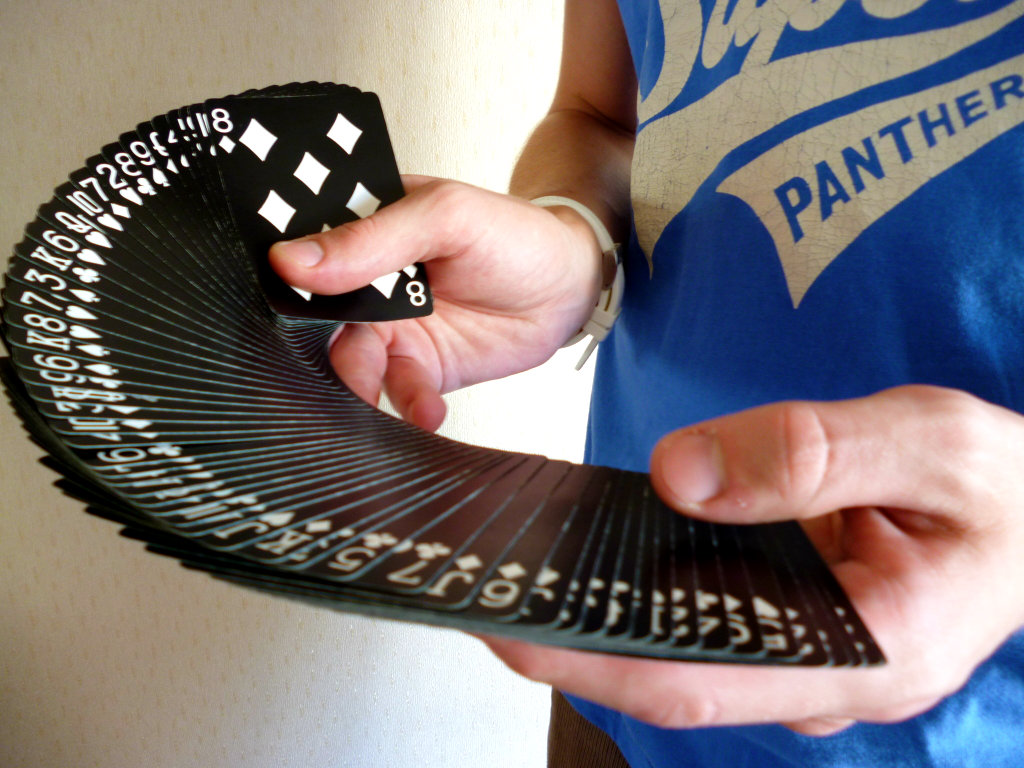A man in a blue t-shirt with a gray or silver pattern, the bottom of which reads "Panther," is holding a fan of playing cards. The cards, all black with intricate white patterns, are spread out face-up, showcasing various values. The most prominent card in the center is the Eight of Diamonds, featuring eight white diamonds and corresponding symbols. The man’s right arm, adorned with a white-banded wristwatch, is bare up to the shoulder, suggesting that the t-shirt might be sleeveless. The scene is set indoors against a white or cream-colored wall, with the person slightly backlit. The cards appear to be shuffled, indicating that the deck is complete and in use.